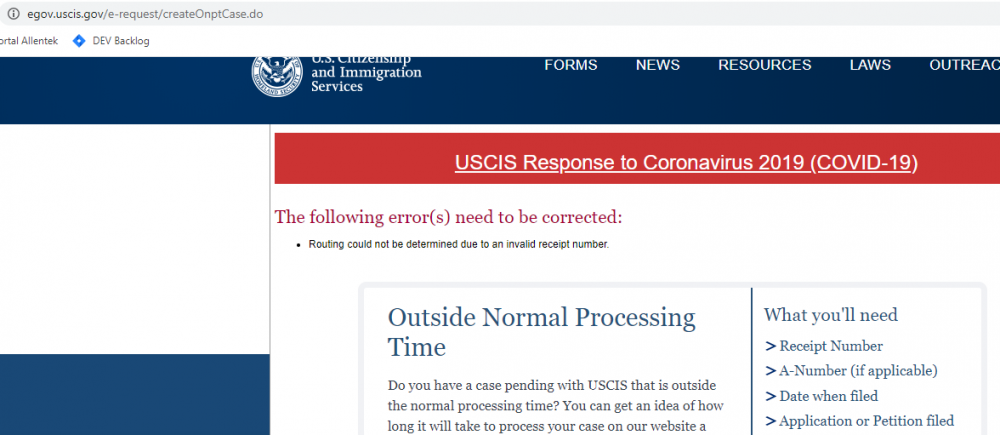This screenshot displays a partially cropped web page from the U.S. Customs and Immigration Service (USCIS) website, capturing a series of user interface elements and messages. At the top, the URL bar is visible, indicating the address "e-gov.usdas.gov/e-request/createONPTCART.e-gov." Below the URL, a noticeable web mark links to an Atlassian Prodigy's DEB backlog. 

The header contains a prominent red alert banner that reads, "USCIS Response to Coronavirus 2019 (COVID-19)," signaling important information regarding pandemic-related updates. Beneath this alert, an error message states: "The following errors need to be corrected. Routing cannot be determined due to an invalid receipt number." This indicates a problem with user-submitted data.

Further down, a card section titled "Outside Normal Processing Time" poses a question to users: "Do you have a case pending with USCIS that's outside the normal processing time?" It offers assistance in estimating case processing durations and lists required information for this inquiry, including a receipt number, A-number (if applicable), filing date, and the type of application or petition. The remainder of this section is partially obscured due to the cropped nature of the screenshot, leaving additional details unreadable.